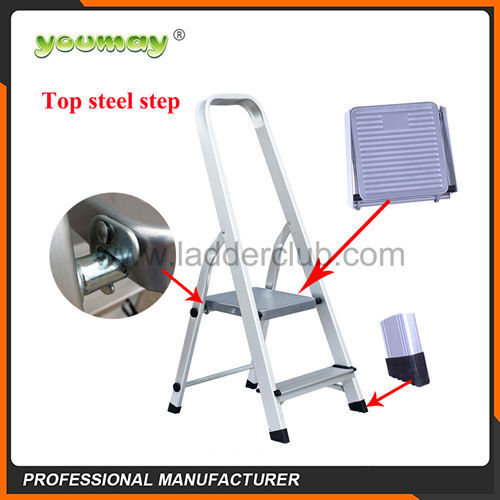The square-shaped image, likely designed for a website, features an instructional diagram for a metal step ladder with two steps, showcased against a white background. The image is framed by a distinct orange and black border. At the bottom of the image, "Capital Print Professional Manufacturer" is displayed in white text on a black backdrop. In the top left corner, bold green text reads "You May," followed by red text stating "Top Steel Step." 

The central focus of the image is a silver-colored step ladder with detailed annotations. Various components of the ladder are highlighted by red arrows and zoomed-in sections. On the left side, an arrow points to the locking mechanism with an enlarged view for clarity. The top right section features an arrow directing attention to the ladder's top step, complete with non-slip lines, supported by an enlarged illustration. The bottom right corner displays another arrow to the ladder's foot, emphasizing the black rubber cap designed to prevent floor scratches and provide stability. This comprehensive and detailed layout is emblematic of product images typically seen on e-commerce websites, providing clear and detailed information for potential buyers.